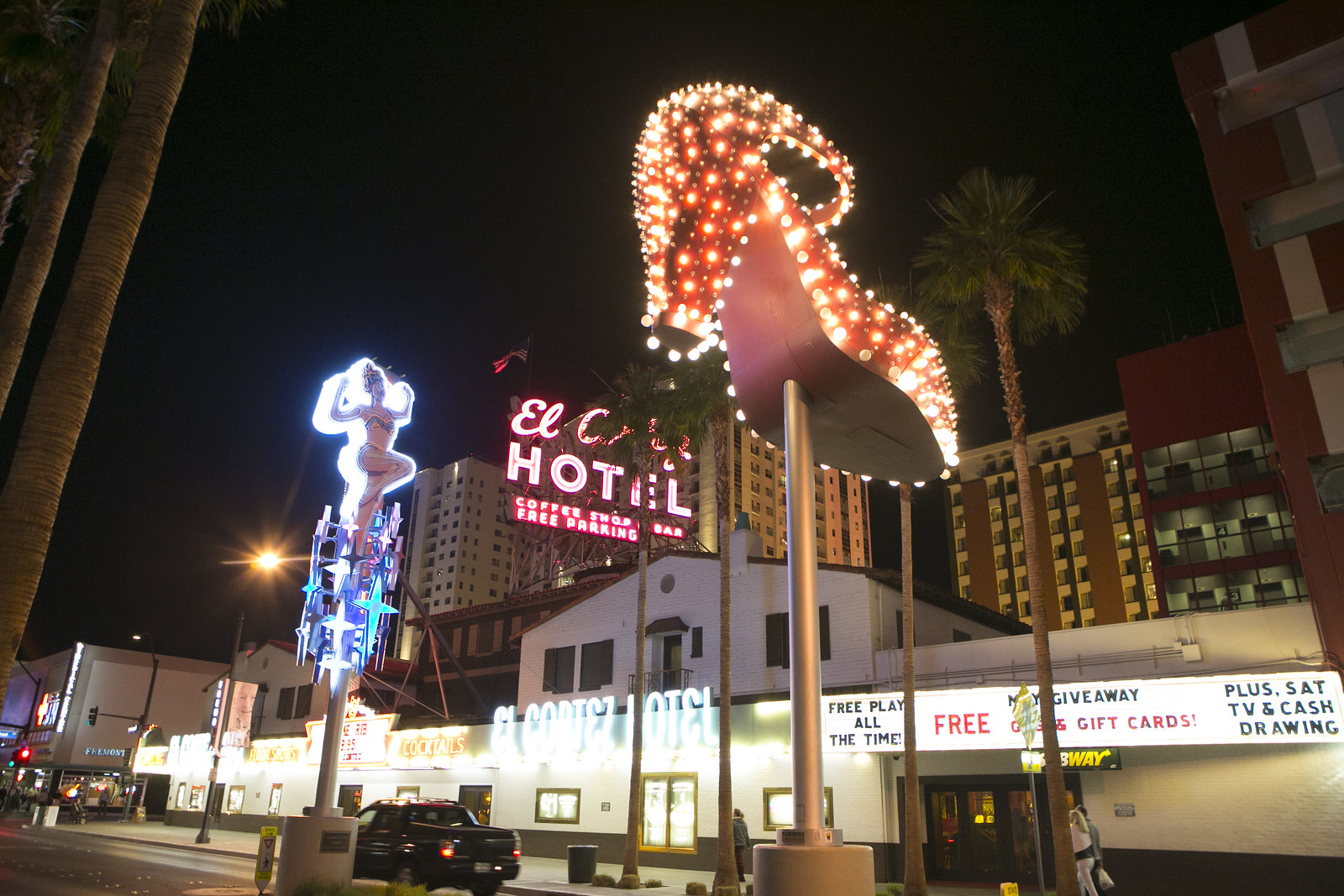This detailed photograph captures the vibrant facade of the El Cortez Hotel and Casino, a central focus within an entertainment complex reminiscent of the Las Vegas Strip. Dominating the scene, the blue neon sign atop the building prominently displays "El Cortez Hotel," with additional text advertising "Free Play All the Time," "Free Giveaway Gift Cards," along with "Satellite TV and Cash Drawing." Below this marquee, a Subway restaurant sign is clearly visible. To the right, a large neon sign in the shape of a brightly lit, strappy high-heeled shoe in pink and yellow adds to the lively ambiance. Adjacent to this, another striking neon sign features a woman in a swimsuit, striking a dancing pose beneath glittering stars, contributing to the festive atmosphere of the street. Pedestrians can be seen strolling along the sidewalk, and a black truck drives by on the road. The overall scene is further animated by various neon lights and signs, including a cocktail bar to the left of the hotel’s signage, all working together to create a quintessential Las Vegas street scene filled with entertainment and dazzling lights.